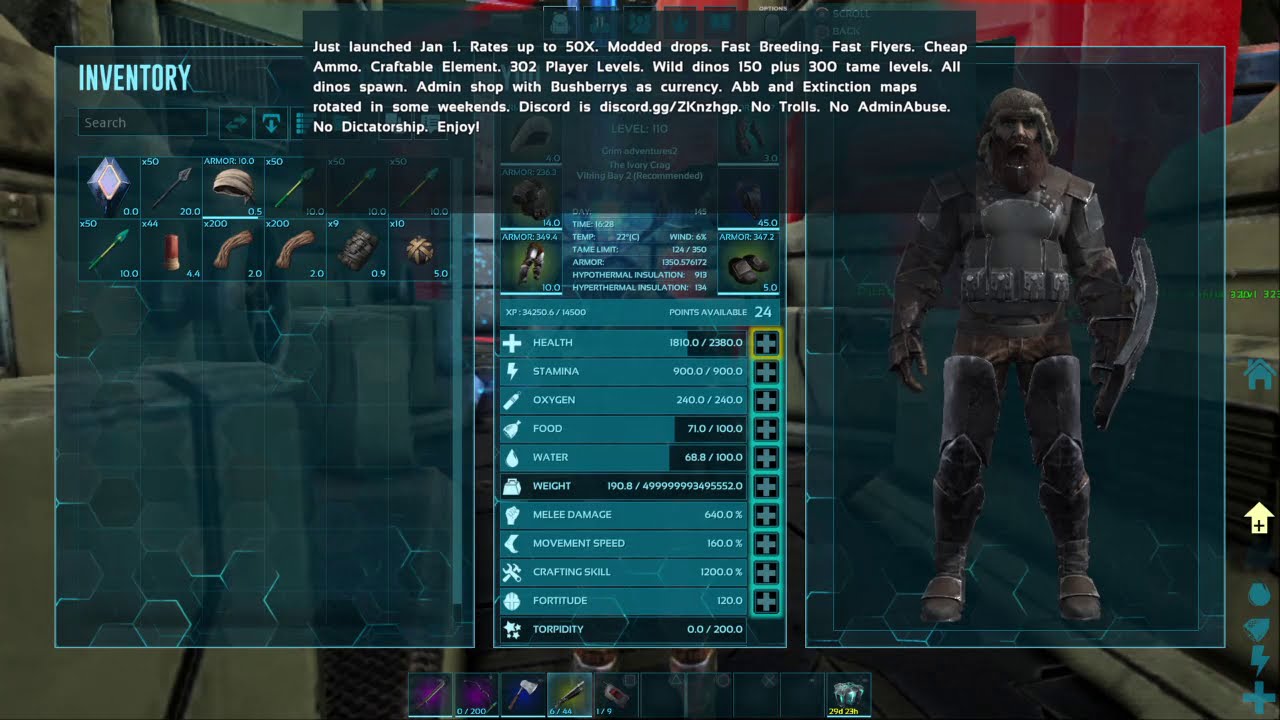The image is a detailed screen capture from a video game focused on a battle scenario. The background displays a faded image of the interior of a space or aircraft, showcasing the backs of some seats and streamlined metal walls. Superimposed on this background is a framed interface with critical game information. 

On the left-hand side of the frame, in a glowing blue font, the word "Inventory" stands out, indicating the section where various items are displayed. The inventory includes icons of items such as a diamond, spears, a turban, something resembling a firecracker, arms or gloves, a mask, and a ball, each neatly arranged in labeled squares. Beneath "Inventory" is a search bar for locating specific items.

In the middle of the frame, a prominent chart lists vital statistics written in white font against blue bars. This chart provides readings for health, stamina, oxygen, food, water, and other essential metrics. Positioned at the top center of the interface is a block of text detailing the game's recent launch on January 1st, emphasizing features like boosted rates up to 50x, modded drops, fast breeding and flyers, cheap ammo, craftable equipment, and other enhancements. Additional information indicates 302 player levels, wild dino levels of 150 plus 300 tame levels, and mentions an admin-run shop using bush berries as currency. The game includes rotating maps, specifically ABB and Extinction, on some weekends. A Discord link (discord.gg/ZKNZHGP) is provided, along with community guidelines such as no trolls, no admin abuse, and no dictatorship.

On the right side of the frame is a character display featuring a male figure clad in green and brown body armor. The character sports a helmet, a long red beard and mustache, and is equipped with a large shield on his left arm. He also wears thigh and knee padding, along with sturdy boots, giving him a battle-ready appearance.